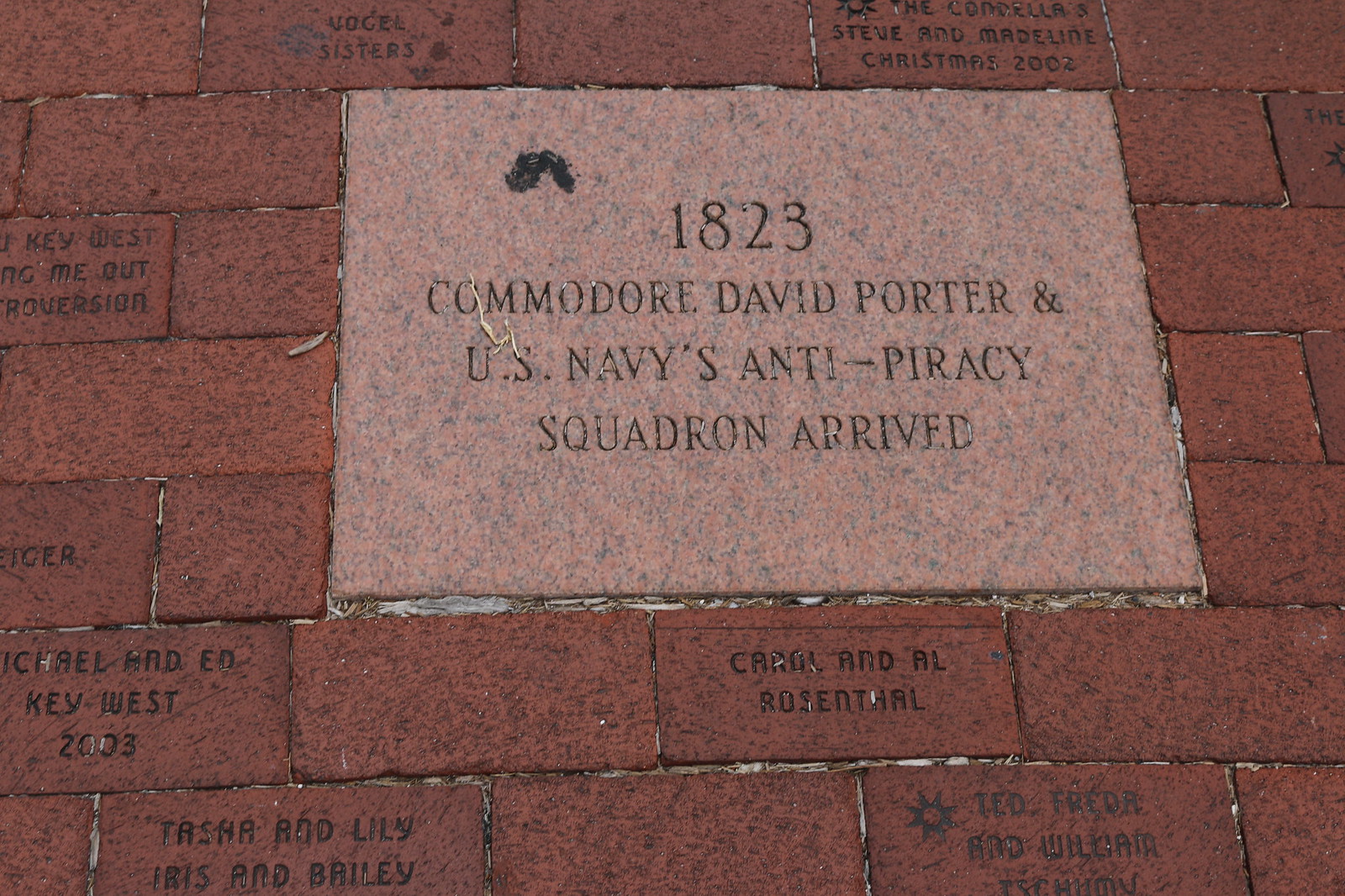The photograph depicts a memorial site consisting of an arrangement of bricks on the ground. At the center lies a prominent, light brownish-pink brick that stands out significantly due to its larger size and lighter color compared to the surrounding dark red bricks. Engraved on this central brick is the inscription: "1823 Commodore David Porter and U.S. Navy's Anti-Piracy Squadron arrived." Encircling this main brick are numerous smaller dark red bricks, each featuring engraved names and messages. Notable inscriptions on these surrounding bricks include "Carol and Al Rosenthal," "Ted Fida," "William," "Tashemi, Tasha, and Lily," "Iris and Bailey," "Key West," "Meowt," "Troversion," "Vogel Sisters," "Michael and Ed Key West 2003," "The Connellas," and "Stephen and Madeline Christmas 2002." The detailed engravings on the bricks provide a poignant reminder of the individuals and events commemorated at this memorial site.